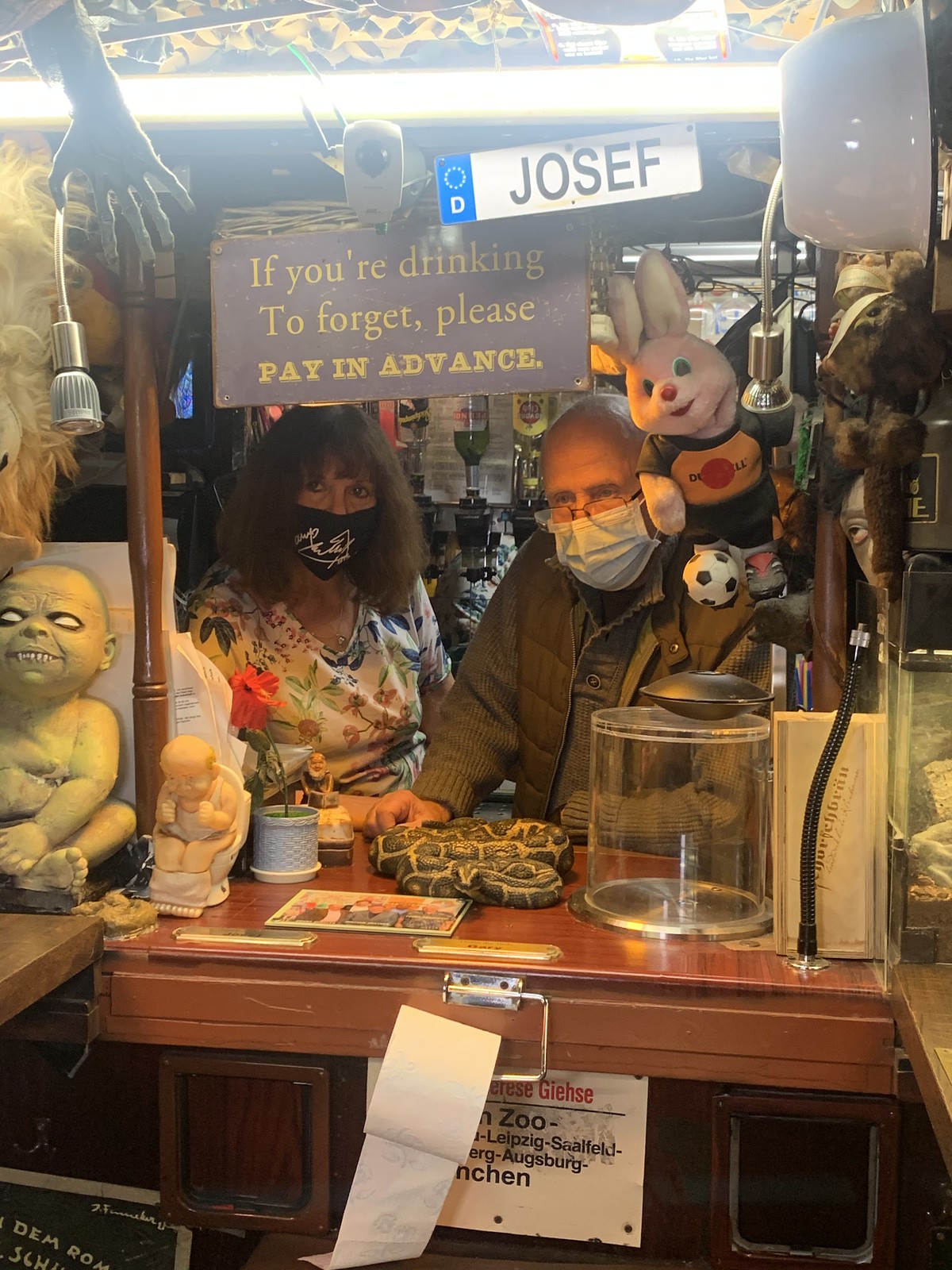The rectangular photograph captures a highly eclectic bar setting with two people behind a cluttered wooden counter. The bar itself appears to be made of maple-colored wood. On the left is a woman with long dark brown, slightly frizzy hair, wearing a black mask adorned with white writing, and a colorful t-shirt featuring multicolored flowers against a white background. To her right stands an elderly, bald gentleman, sporting glasses, a blue disposable medical mask, a brown knit sweater, and a brown vest.

A bizarre array of items surrounds the pair. On the counter is a live green snake, coiled and resting. Next to the snake is a clear display case, which appears empty, and a white pot holding a red flower. Various eccentric collectibles are scattered around, including a toy of a man sitting on a toilet, a rubber hand reminiscent of a zombie, and a dancing flower.

Above them, a sign humorously reads, "If you're drinking to forget, please pay in advance," while another sign simply states "Joseph." To the right of the signs, a security camera keeps watch. Hanging nearby is a stuffed pink bunny and, further left, a creepy, shirtless doll with a distorted face, resembling a "Buddha baby." Among these numerous mismatched items, a toilet paper holder with a roll of toilet paper dangles off the bar's edge, adding to the chaotic ambiance. Additionally, liquor taps are visible behind the counter, highlighting the bar's primary function amid the chaos.